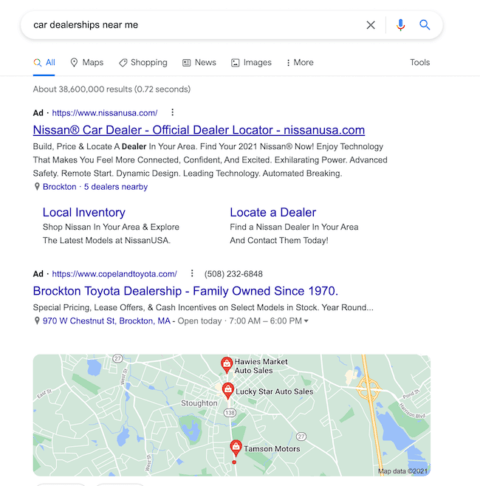This is a detailed screenshot of a Google search results page for the query "car dealerships near me." The search yielded approximately 38,600,000 results in 0.72 seconds. The visible portion of the results includes two advertisements at the top. 

The first ad is from Nissan, labeled as the "Official Dealer Locator" and linked to NissanUSA.com, suggesting it directs users to the general U.S. Nissan site.

The second ad is for the Brockton Toyota dealership, a family-owned business since 1970. The URL CopelandToyota.com indicates it’s a specific dealership located at 970 West Chestnut Street, Brockton, Massachusetts. The operational hours listed show that it is open today from 7 a.m. to 6 p.m.

Below these ads, there's a visible portion of a map featuring pinned locations of nearby car dealerships. The map highlights three specific businesses: Holley's Market Auto Sales, Lucky Star Auto Sales, and Tamsen Motors.